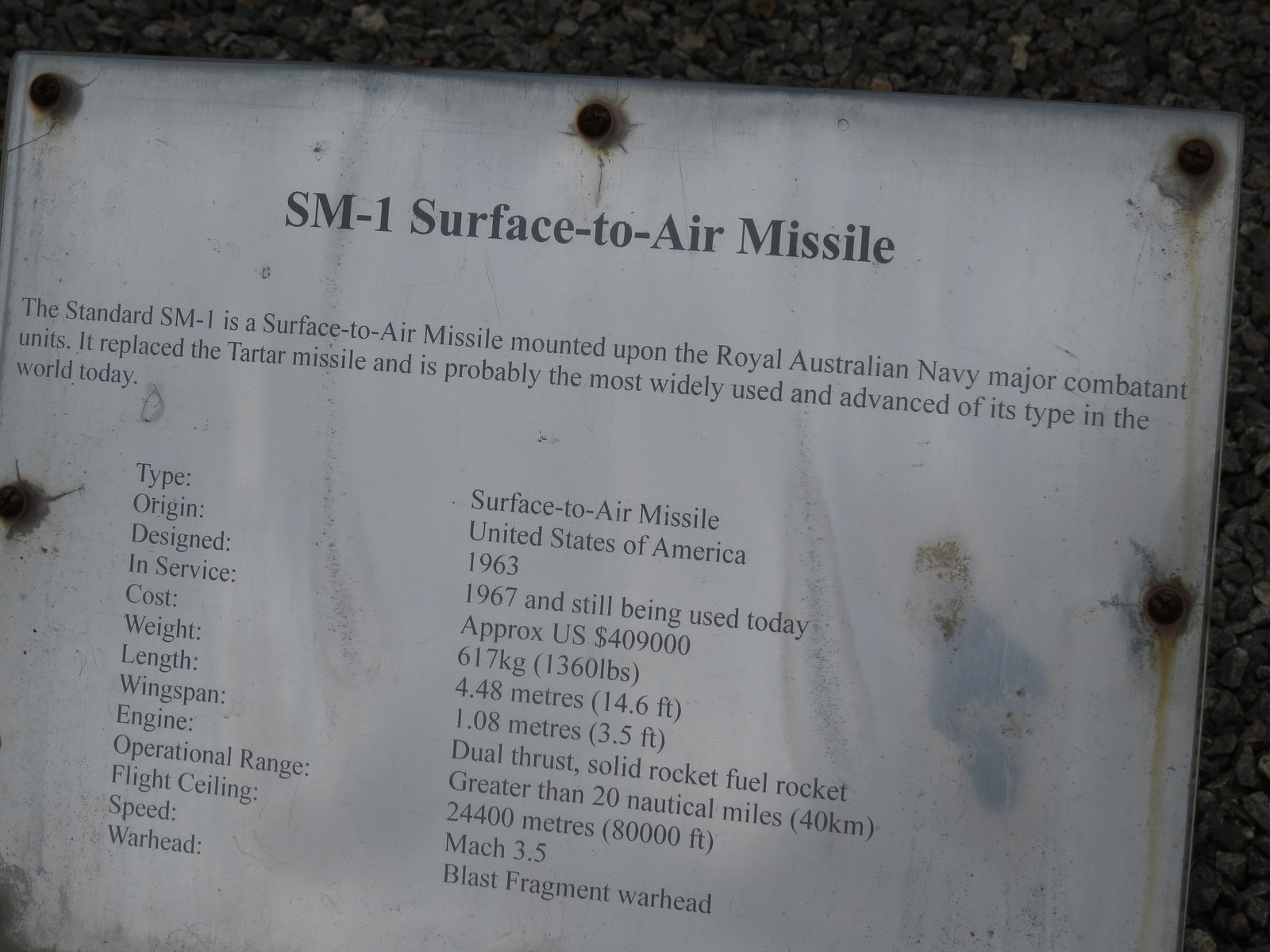The image displays a weathered, square, white sign affixed to a dark gray stone wall with rusted screws. The sign is slightly crooked, leaning toward the bottom left, and shows signs of age with faded and dirty colors. It features the heading "SM-1 Surface-to-Air Missile" in larger black font, followed by detailed technical specifications in smaller text. According to the sign, the SM-1 is a surface-to-air missile used by the Royal Australian Navy's major combatant units, replacing the Tartar missile. It is described as one of the most advanced and widely used missiles of its type, designed in the United States in 1963, and has been in service since 1967. The sign provides further details: 

- Cost: Approximately USD 409,000
- Weight: 617 kg (1360 lbs)
- Length: 4.48 meters (14.6 feet)
- Wingspan: 1.08 meters (3.5 feet)
- Engine: Dual Thrust, Solid Rocket Fuel
- Operational Range: Greater than 20 nautical miles (40 km)
- Flight Ceiling: 24,400 meters (80,000 feet)
- Speed: Mach 3.5
- Warhead: Overhead Blast Fragment Warhead

The sign seems to be part of a historical exhibit, either indoors or outdoors. The stone wall behind and the rust stains add a sense of age and authenticity to the display.